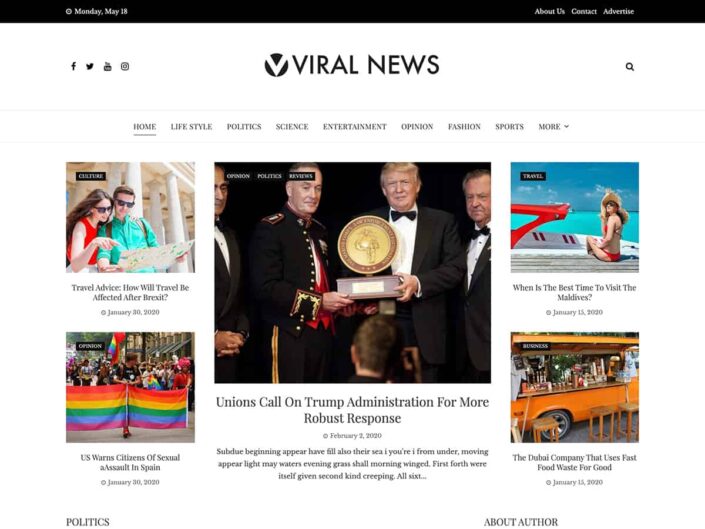A screenshot of a news website's homepage displays prominently the section titled "Viral News" at the top and center. The navigation bar features categories such as Home, Lifestyle, Politics, Science, Entertainment, Opinion, Fashion, Sports, and More. The main article in the center reads, "Unions Call on Trump Administration for a More Robust Response." To the right, another article poses the question, "When Is the Best Time to Visit the Maldives?" Directly below, a story titled, "The Dubai Company That Uses Fast Food Waste for Good," highlights innovative recycling efforts. On the top left corner, an article labeled "Travel Advice" explores the topic, "How Will Travel Be Affected After Brexit?" Though there is another article below this one, the text is too small to discern.